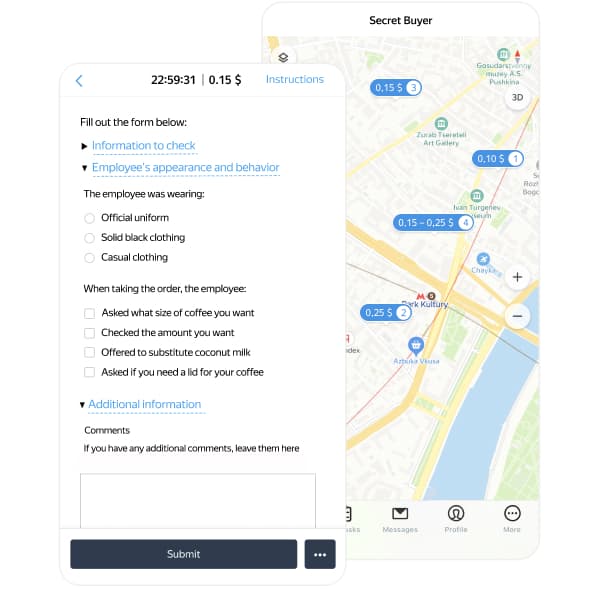The image is split into two distinct sections placed side by side. 

On the left side, the screenshot has a white background adorned with a combination of blue and black text. At the top, there's a black arrow pointing to a timestamp in black text reading "$22.59.31." Below it, another black text displays "$0.15" followed by the word "instructions." Below this header, there are instructions that read, "Fill out the form below, information to check, employees, appearance, and behavior," each accompanied by a black arrow.

Further down, the form prompts with, "The employee was wearing," and offers three checkbox options within white circles: "Official uniform," "Solid black clothing," and "Casual clothing."

Next, there is another section titled, "When taking the order, the employee," followed by several white checkboxes with the options: "Asked what size coffee you want," "Check the amount you want," "Offered to substitute coconut milk," and "Asked if you need a lid for your coffee."

Following this, a segment marked "Additional information" with a black down arrow, and a section for "Comments" invites the user to leave additional remarks in a provided white box. Beneath this input field, there are two buttons: one black box with white text that reads "Submit," and another black box featuring some dots.

The right side of the image resembles a map interface, possibly from Google Maps or Apple Maps, displaying a mixture of tan, gold, and green hues to denote different land areas. Streets are highlighted in yellow, and various prices such as "$0.15," "$0.10," "$0.15 to $0.25," and "$0.25" appear in white circles.

Within the map, small blue and white shopping icons are scattered across, alongside blue, green text, and a prominent red arrow. A plus (+) and minus (-) sign within a circle, likely for zoom control, are also visible. At the very bottom of this section is a submenu containing tabs labeled “messages,” “profile,” and “more,” providing additional navigation options.